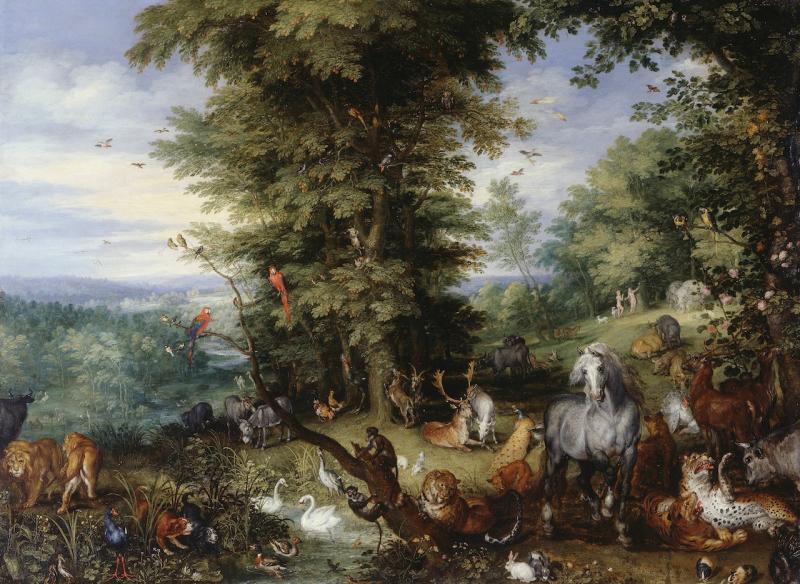This detailed Renaissance-era painting, likely from the 1500s or 1600s, vividly depicts the Garden of Eden. Set on a sprawling hillside with dense forests that extend into the distance, the scene is teeming with diverse wildlife. In the foreground, a variety of animals coexist harmoniously in a secluded clearing amidst tall, thick trees. Among them, red and blue parrots perch on tree branches, small monkeys swing nearby, and diverse birds like swans, doves, and geese populate the scene. Predators and prey such as leopards, dogs, and lions lie in close proximity, alongside more docile creatures like elk, deer, and a majestic white horse. Additional fauna include a bison on the left and exotic animals like a rhinoceros and a dark gray horse. Far in the background, almost hidden from immediate sight, Adam and Eve stand beside a tree, with the woman reaching up, suggesting the moment of temptation with the forbidden fruit. The color palette of the painting is rich and varied, featuring hues of yellow, white, blue, black, red, green, gray, and brown, adding depth and vibrancy to the serene yet intricate tableau.